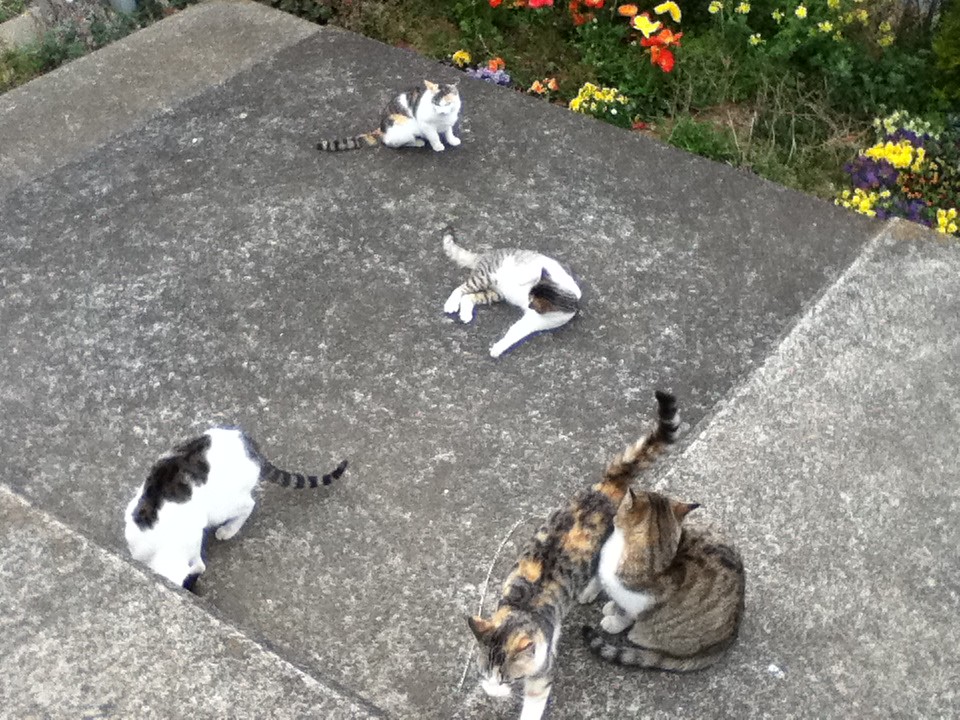The image depicts a backyard scene centered on a gray concrete porch. Five different cats with varying fur colors are scattered across the slab. There are three predominantly white cats, including one with a large gray patch on its back and another with black spots and a gray tail. Two other cats feature more intricate patterns: one is a calico with a mix of colors, and the other has gray stripes along its body. The calico cat is walking past another cat that is poised gracefully, sitting with its tail wrapped around its body. This cat has a white breast and a mix of gray, black, and tan fur. Two cats sit close together in the bottom right corner, seemingly rubbing up against one another. A flower garden filled with vibrant red, yellow, purple, and white flowers encircles the porch, adding a colorful contrast to the scene. The cats are engaged in various activities: lounging, walking, and sitting, making the scene lively and charming.